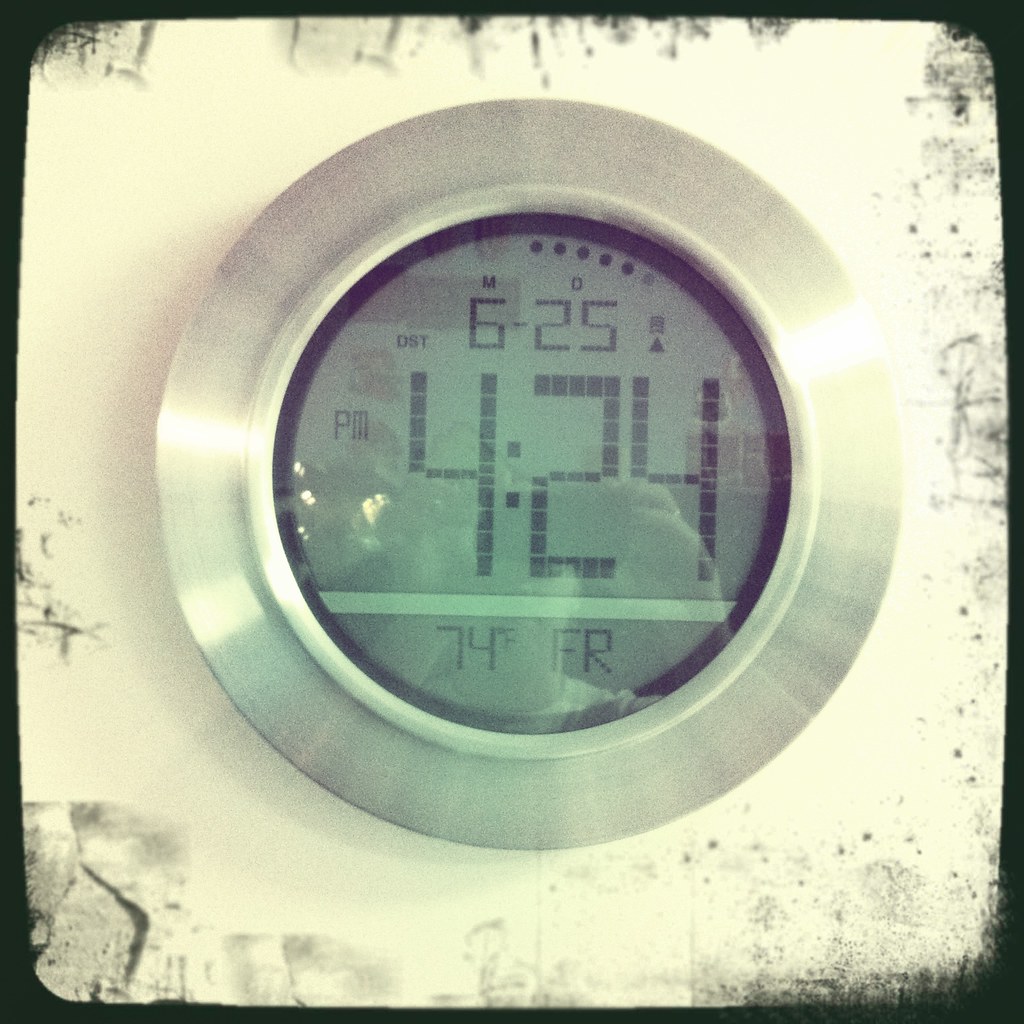The digital clock hangs on a pristine white wall, encased in a sleek stainless steel circular frame. The display area of the clock has an aged, bluish-gray tint, characteristic of older digital timepieces. At the very top of the display, the day of the week is indicated by an "M" for Monday. Directly below this, the date is shown as "6" for the month and "25" for the day. Beneath the date, the time is displayed prominently as "4:24 PM," with a thin white line beneath the digits. Below the line and to the left, the temperature is shown as "74 degrees," with an "F" for Fahrenheit and an "R" immediately to its right. Upon close inspection, the reflective surface of the clock reveals the faint reflection of a person's head and several indistinct reflections on either side.